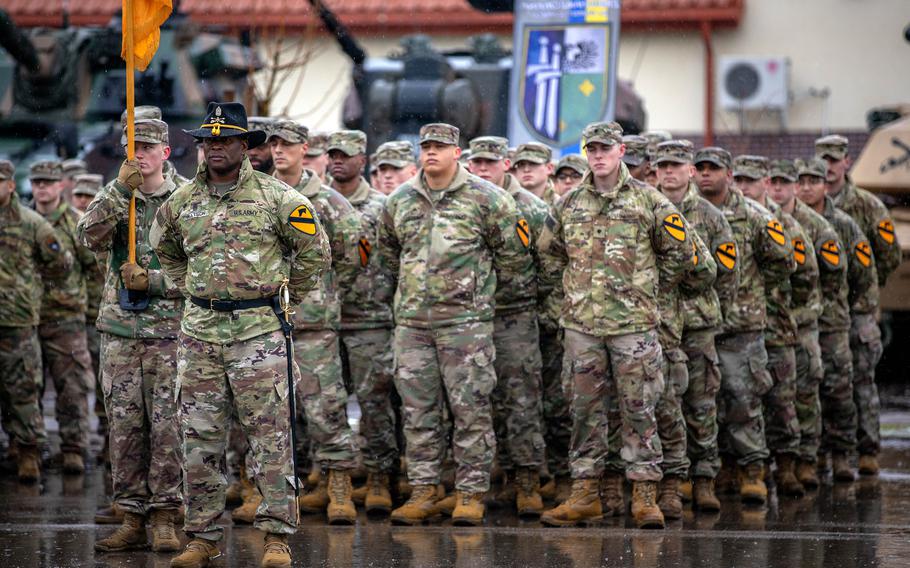This full-color, horizontally rectangular photograph captures a meticulously posed scene of military troops in formation, taken indoors under artificial lighting. Dominating the foreground is an African-American gentleman dressed in fatigues and sporting a distinct black cavalry hat adorned with a yellow ribbon. He wears a sword on his belt, adding to his commanding presence. Slightly behind him, another soldier holds a prominent yellow flag.

The formation consists of several orderly rows of soldiers, all clad in camouflage uniforms and brown boots, indicating their readiness and discipline. Each soldier's right arm proudly bears a yellow patch with a black diagonal stripe and a black symbol, likely denoting their specific division. The troops stand at ease, reinforcing the posed nature of the photograph.

In the distant background, to the left, is another flag featuring a design with crossed swords. Although the photograph is taken indoors with no detailed background visibility, the overall scene is filled with an air of military precision and unity.